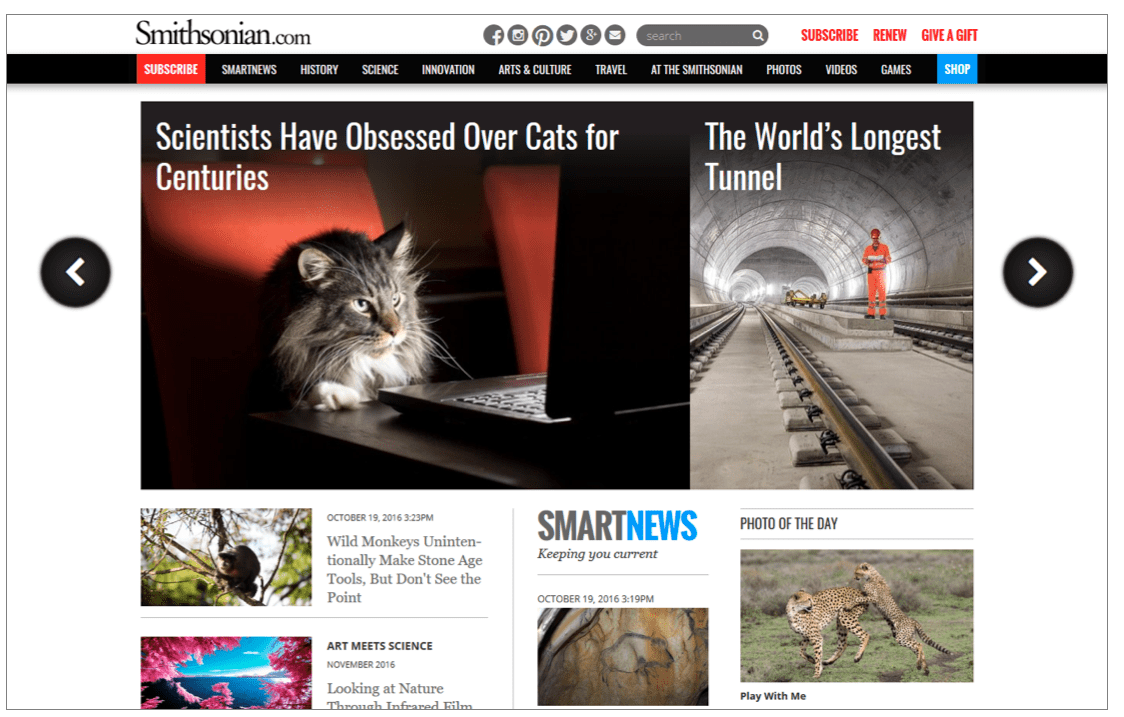This is a detailed caption for the given image:

The screenshot showcases The Smithsonian website, prominently featuring 'smithsonian.com' on a white border at the top. Social media icons for Facebook, Instagram, Pinterest, Twitter, Google, and an email icon are aligned next to a search bar. To the right, in red font, are the options 'Subscribe,' 'Renew,' or 'Give a Gift.' Below, a black border houses a red button with white lettering that reads 'Subscribe.' The navigation bar lists categories including Smart News, History, Science, Innovation, Arts & Culture, Travel at the Smithsonian, Photos, Videos, Games, and Shop. 

The headline section below introduces intriguing articles: "Scientists Have Obsessed Over Cats for Centuries," featuring an image of a cat gazing at a laptop; "The World's Longest Tunnel"; and "Wild Monkeys Unintentionally Make Stone Age Tools but Don’t See the Point." An enticing section, "Art Meets Science: Look at Nature Through Infrared Film," follows. The Smart News section aims to keep readers current, below which the "Photo of the Day" showcases an image titled "Play with Me," depicting two leaping leopards. One leopard is mid-air, seemingly leaping at the rear of the other, which is also airborne and glancing backward at its companion.